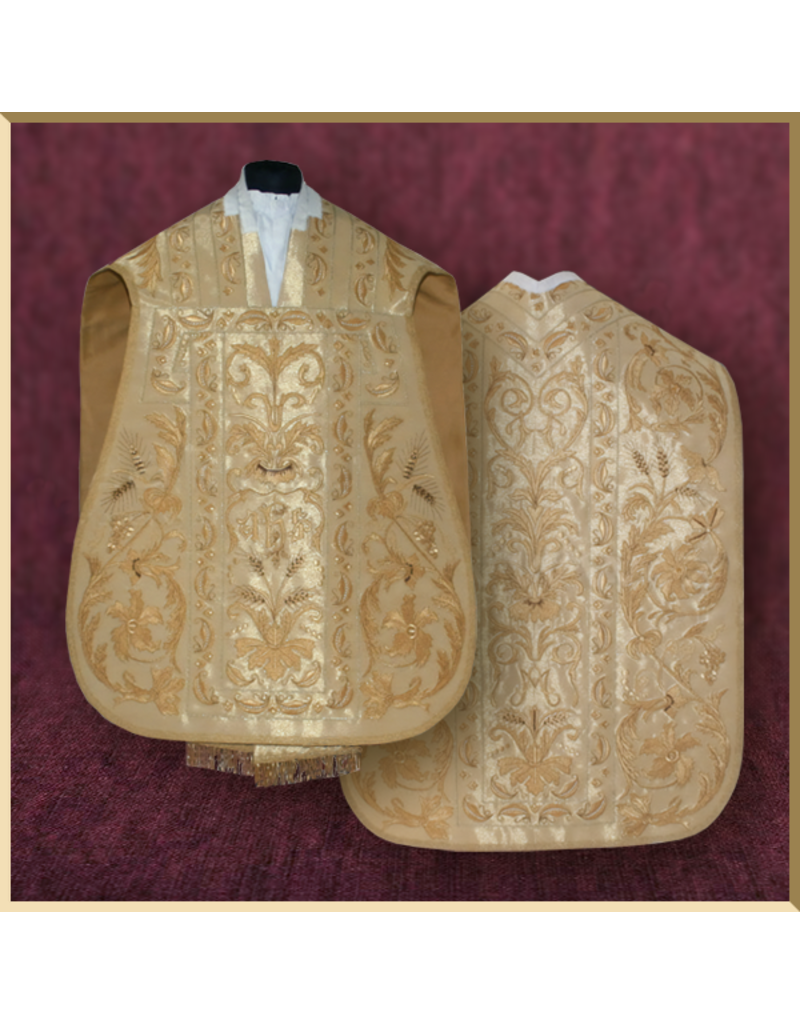This image is a perfectly square photograph with a gold border surrounding a deep maroon interior. Within the central area, the image showcases two intricately designed vests, both appearing splendid in gold material, rich with ornate floral and leaf patterns.

In the upper left section of the image, the front of the vest is prominently displayed. It features a V-shaped neckline with detailed white trim around the neck. This section is meticulously laid over a portion of the back of the vest, which occupies the lower right part of the image. The back of the vest mirrors the front in its elaborate decoration but is further enhanced by what seems to be intricate argyle and flowery designs, also trimmed with white around the neck.

The positioning creates a slight overlay where the front piece covers about a third of the back piece, creating a layered effect that highlights both sides. The vests appear to be mounted on an unseen form, suggesting a mannequin, to provide structure as there are no visible arms, legs, or a head. The depth of field adds visual interest, as the maroon background fades into a blur at the top while remaining in focus at the bottom.

Overall, the image exudes a sense of historical elegance, showcasing the affluent design typical of centuries-old attire, meant to be admired both for its craftsmanship and ornate detailing.